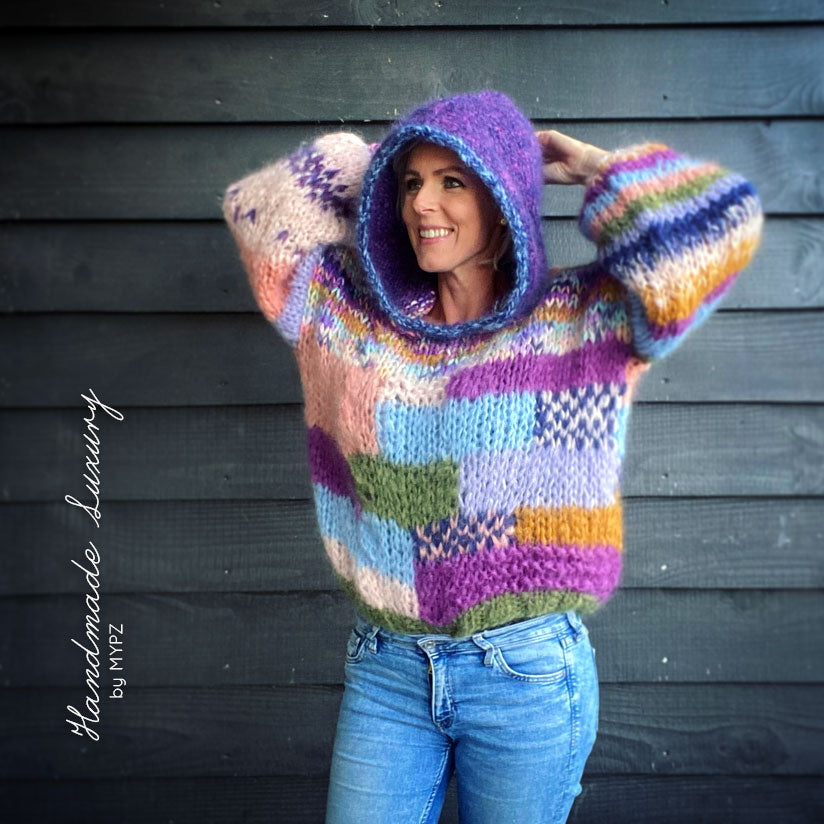A captivating advertisement showcases a smiling Caucasian woman standing in front of a rustic wood wall reminiscent of a cabin’s exterior, with charcoal grey horizontal planks. The focal point is her vibrant, thick knitted sweater composed of rectangular sections in shades of purple, blue, green, orange, and white. The sweater features a distinctive hood that is purple with a blue trim, pulled over her head, partially obscuring her short blonde hair. She is wearing mid-blue jeans that are visible just above her knees. The woman stands with her hands behind her head, looking off towards her right, displaying a bright, toothy smile. Vertically printed on the lower left side of the image in white cursive text, it reads “Handmade Luxury,” with “By MYPZ” written below in a smaller white font.